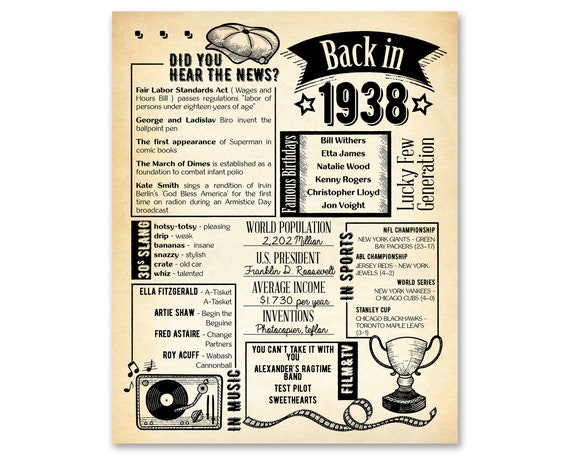**Poster from 1938**

In the upper right-hand corner, bold black text reads "Back in 1938." The news-style poster shares significant events, notable births, popular slang, and cultural highlights from the year.

**Major Events:**
- **Legislation**: Introduction of the Fair Labor Standards Act, setting regulations for wages and hours and labor restrictions for individuals under 18.
- **Innovations**: George and Ladislav invent the ballpoint pen.
- **Entertainment**: The first appearance of Superman in comic books.
- **Health**: Establishment of the March of Dimes foundation to combat infant polio.
- **Music**: Kate Smith performs Irving Berlin's "God Bless America" for the first time on the radio during the Armistice Day broadcast.

**Famous Birthdays:**
- Bill Withers
- Etta James
- Natalie Wood
- Kenny Rogers
- Christopher Lloyd
- Jon Voight

**Popular Slang:**
- **Hotsy-totsy**: Attractive, pleasing
- **Palooka**: A clumsy or uncouth person
- **Drip**: A dull or weak person
- **Bananas**: Insane
- **Snazzy**: Stylish
- **Crate**: An old car
- **Whiz**: Talented person

**Music:**
- Ella Fitzgerald: "A-Tisket, A-Tasket"
- Artie Shaw: "Begin the Beguine"
- Fred Astaire: "Change Partners"
- Roy Acuff: "Wabash Cannonball"

**Film and TV:**
- "You Can't Take It With You"
- "Alexander's Ragtime Band"
- "Test Pilot"
- "Sweet Hearts"

**Additional Facts:**
- **World Population**: 2.2 billion
- **U.S. President**: Franklin D. Roosevelt
- **Average Income**: $1,730 per year
- **Inventions**: Photocopier and Teflon

The poster captures the essence of 1938, depicting a vibrant snapshot of historical milestones and cultural moments.